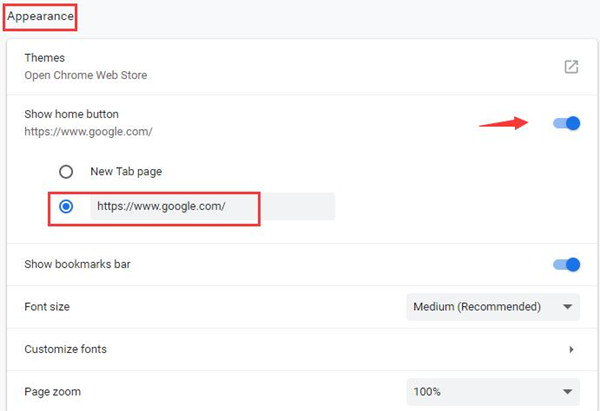The image is a screenshot taken from a device, showcasing a settings page likely from a web browser, specifically focusing on the "Appearance" settings. At the top, the word "Appearance" is prominently highlighted with a red rectangle around it. On the left side of the page, there's a column with a list of options. The first option is "Themes", followed by a link labeled "Open Chrome Web Store."

Below this, there is an option labeled "Show home button" with an accompanying URL starting with "https://". Beneath this URL, there are two selectable options: "New Tab page" and the same "https://" URL. The user has selected the latter, indicated by a blue circular marker, and this area is further highlighted by another red rectangle.

To the right, two switch sliders are visible, both set to "on". These switches are visually represented by blue sliders with blue dots positioned to the right. A red arrow points directly at the top slider, highlighting its association with the "Show home button" setting.

Further down the page, there are options to adjust the font size and customize fonts, as well as a "Page Zoom" feature currently set at 100%, with a drop-down menu to modify this setting if necessary.